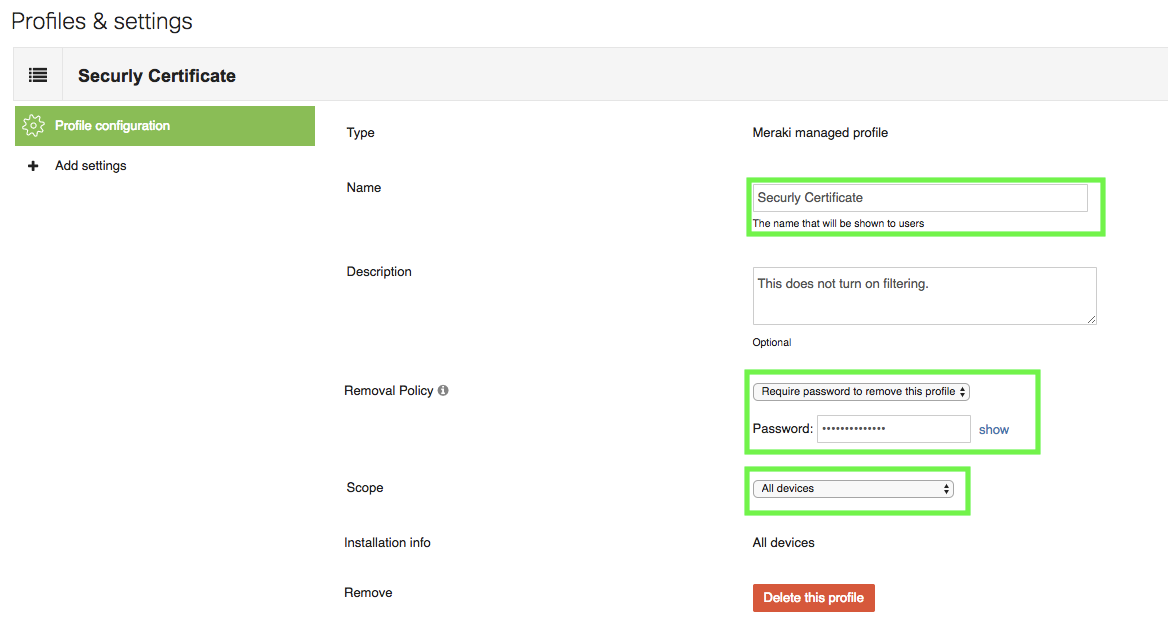This image displays a "Profiles and Settings" page. The title "Profiles and Settings" is prominently featured at the top left in black text set against a white or light gray background.

Directly beneath the title, a gray bar spans the width of the page. This bar is divided into three sections featuring menu icons in dark black text. To the right of these icons, bold black text reads "Secure Lease Certificate."

Below this gray bar, the page returns to a white background and is subdivided into three sections: left, middle, and right.

- **Left Section:** This area is dedicated to widgets. One widget, highlighted in green, is labeled "Profile Configurations" in white text. Below it, there is an option labeled "+ Add Settings."
  
- **Middle Section:** This part appears to be where users can type in information. It features text fields and labels, including "Type," "Name," "Description," "Removal Policy," and a small eye icon, which likely allows for additional options. It is also divided into subsections labeled "Scope," "Installation Info," and "Remove," although none of these fields are currently filled in.

- **Right Section:** This area displays the profile screen. At the very top, it reads "Meraki Managed Profile." Below, in a user-highlighted green rectangle, it states "Secure Lease Certificate" as the name shown to users. A dialog box below that contains the text, "This does not turn on filtering." Additional settings follow, labeled "Optional," "Require Password to Remove this Profile," and "Password," with a password-input box and a "Show" option next to it. Further down, another green label reads "All Devices." At the very bottom of this section, there is a red hyperlink box labeled "Delete this Profile."